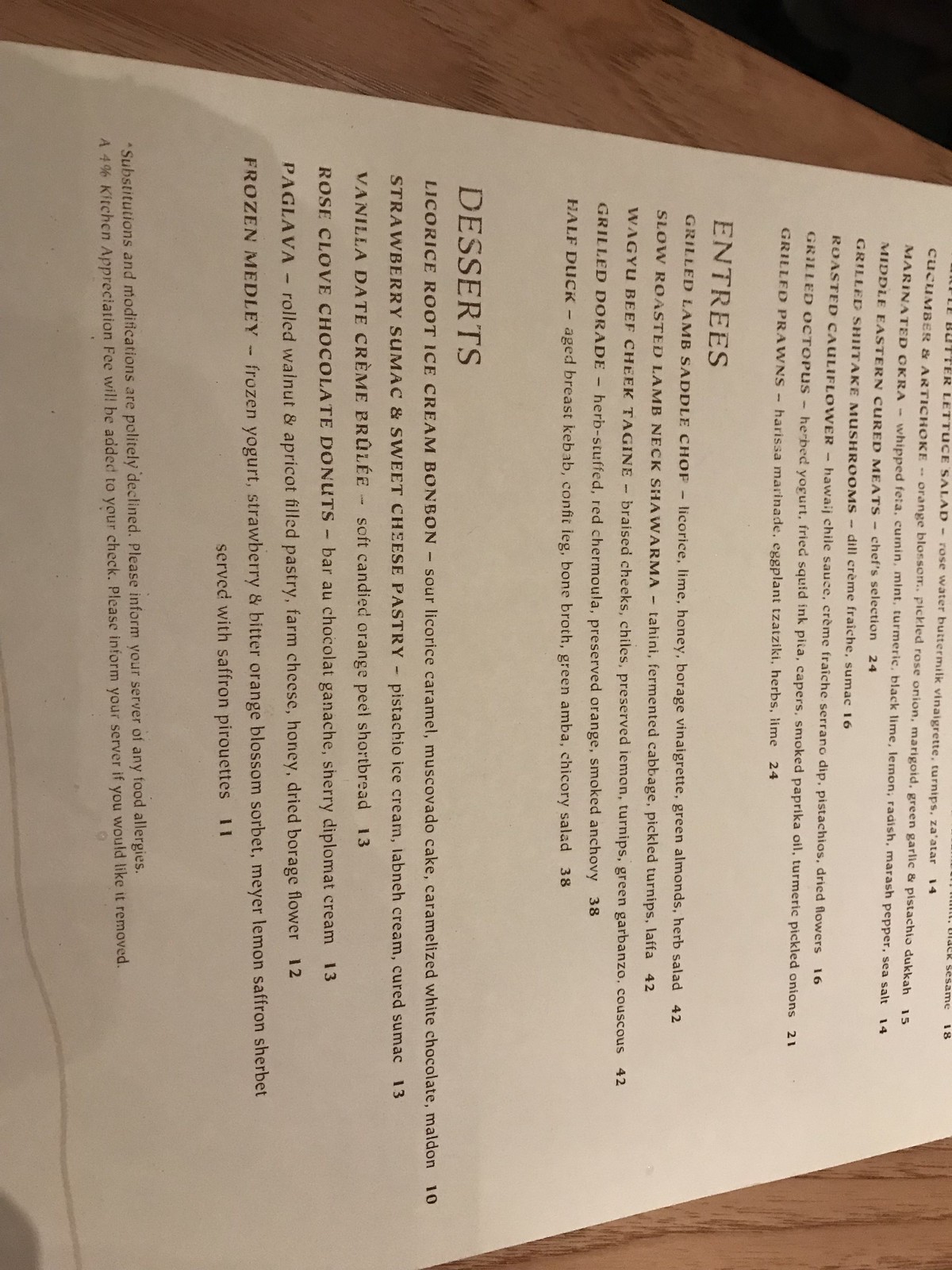The image displays a white menu, with its text oriented incorrectly by being rotated 90 degrees to the right, making the text vertical. The menu is placed on a wooden surface at the bottom of the image. The menu lists a variety of dishes under categories such as appetizers, entrees, and desserts. The appetizers include marinated orca, grilled shiitake mushrooms, and roasted cauliflower. Under entrees, there are options like Middle Eastern cured meats, grilled octopus, grilled prawns, grilled lamb saddle chop, slow-roasted lamb neck shawarma, wagyu beef cheek tagine, and grilled dory. The dessert section offers tantalizing treats like licorice root ice cream bonbon, strawberry sumac and sweet cheese pastry, vanilla date crème brûlée, rose clove chocolate donuts, a dish intriguingly named “peg lava,” and a frozen medley. The black text is printed on the white paper, contrasting sharply against it.